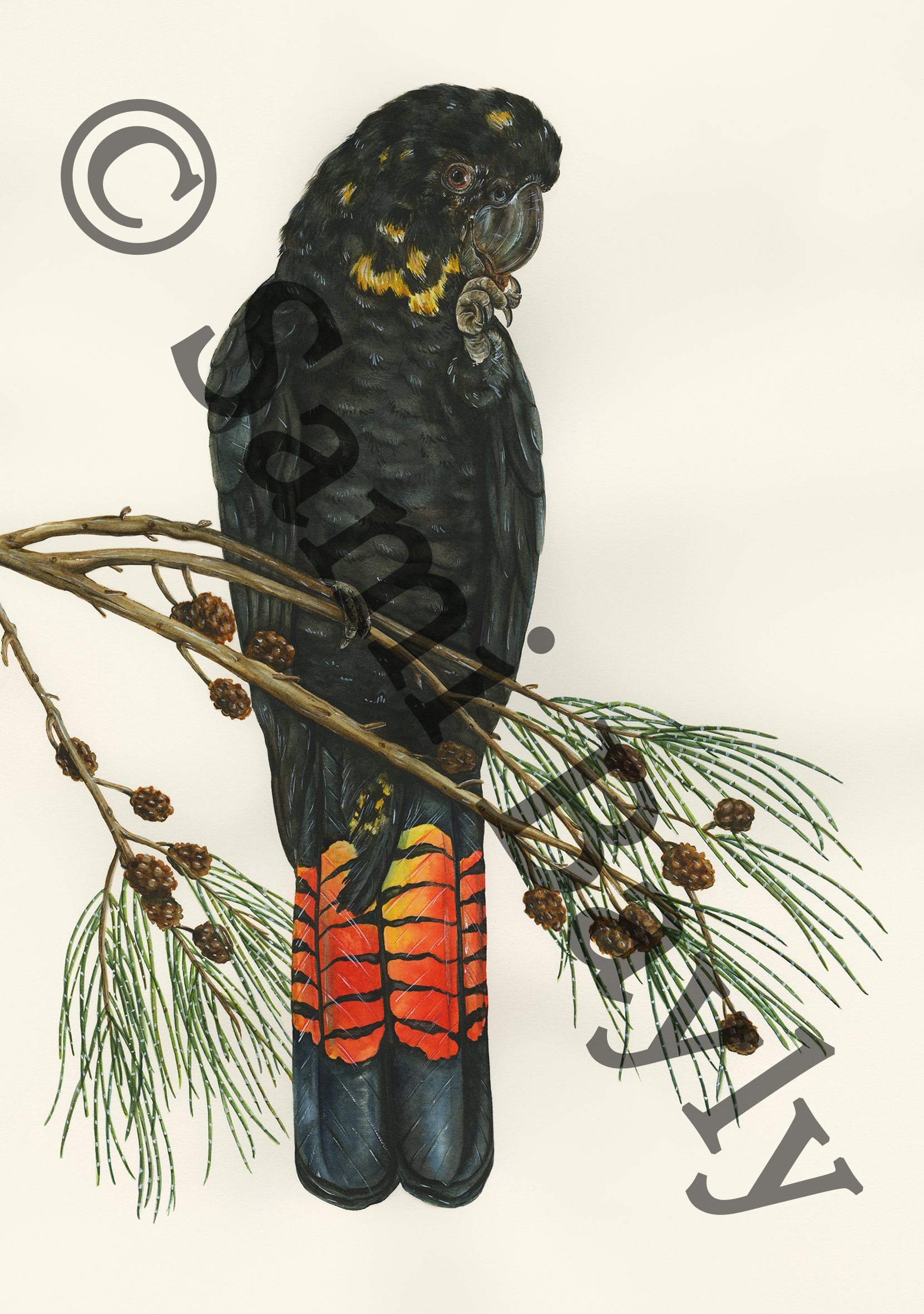The image displays a detailed artwork of a bird perched on a fir tree branch, complete with tassels and tiny pine cones. The bird, primarily black, resembles a parrot with its beak and curved head turned over its right shoulder, allowing one eye and part of the beak to be visible—possibly holding something. Noteworthy is its tail featuring an orange and yellow striped pattern. The background is a tan shade, and a diagonal, transparent watermark across the image from the upper left to the lower right corner reads "© Sammy Bayly" in dark gray lettering, indicating the artist's name. The artwork is non-digital, possibly painted or printed, and the bird appears to be exotic, potentially hailing from South America.